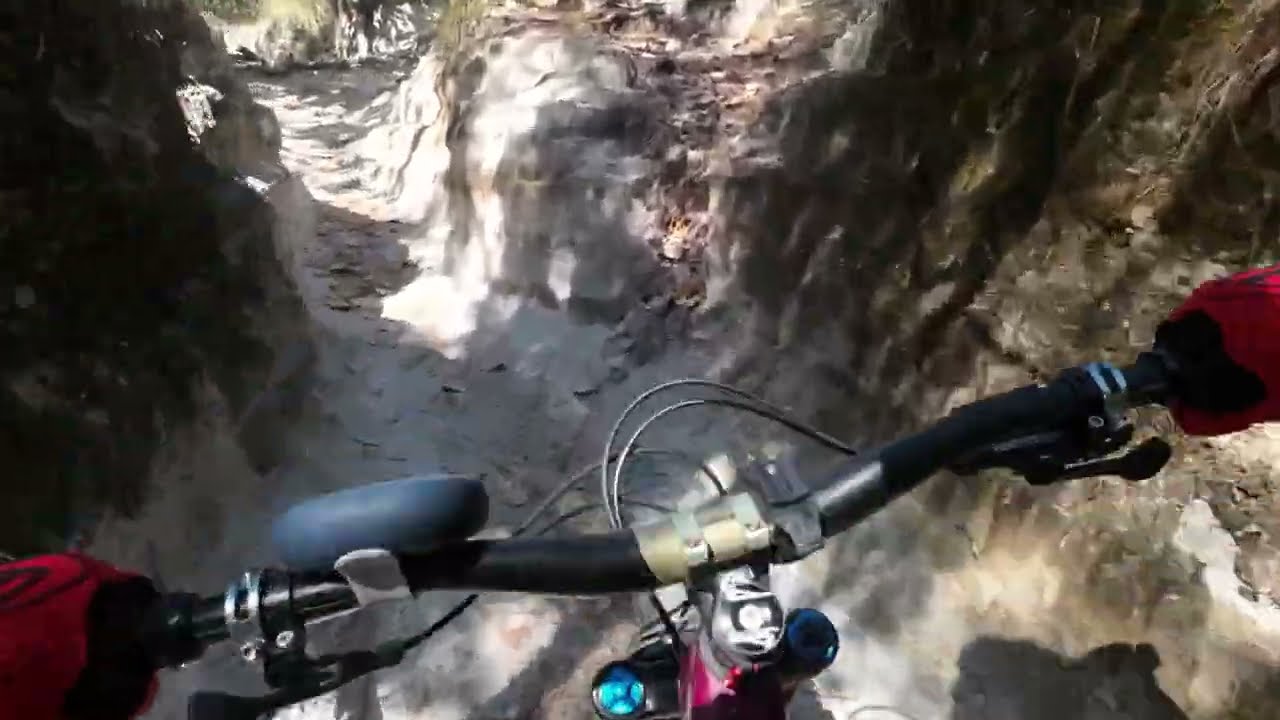The image depicts a first-person view from a mountain biker's perspective as they navigate a rugged outdoor trail. The rider is wearing red gloves, clutching black handlebars that are equipped with grips and various attachments. The trail is set in a rocky canyon with imposing rock formations rising on both sides. The terrain comprises a mix of white and gray rocks, with some sections marked by green moss. The ground underneath is a blend of beige, white, and brown tones. The sun illuminates the scene, casting light over the barren, stone-filled landscape. Ahead of the biker, who is focused on steering through a gap in the canyon walls, lies a large white boulder, setting the course through this striking natural path. Cables from the bike are visible, emphasizing the technicality of the ride in this harsh, scenic environment.